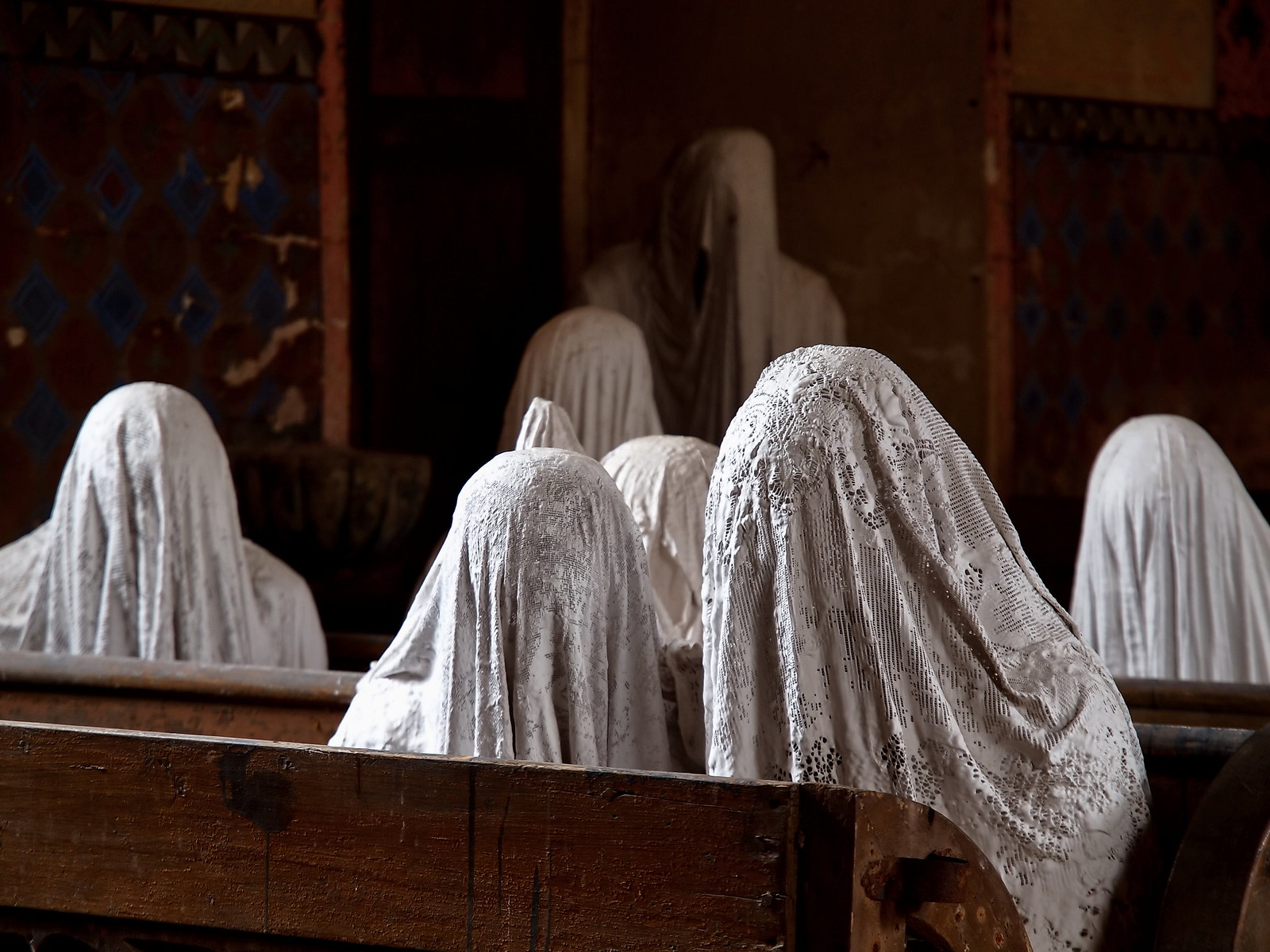In this eerie, undated photograph set in a church, seven figures are seated in wooden pews, all enveloped in various white lace or dowry-like cloths that completely obscure their faces. The setting is marked by wooden walls and pews, bathed in light that highlights the intricate lace patterns of their coverings while leaving the background in shadow. In the foreground, two individuals sit together in the closest pew, with the person on the right noticeably larger, possibly indicating a parent and child. Another pair sits in the next pew, followed by a trio of figures further back, including one standing figure indistinguishable as either a person or a statue, also draped in the same fabric. The solemn air suggests a deep contemplation or prayer amongst the shrouded figures.